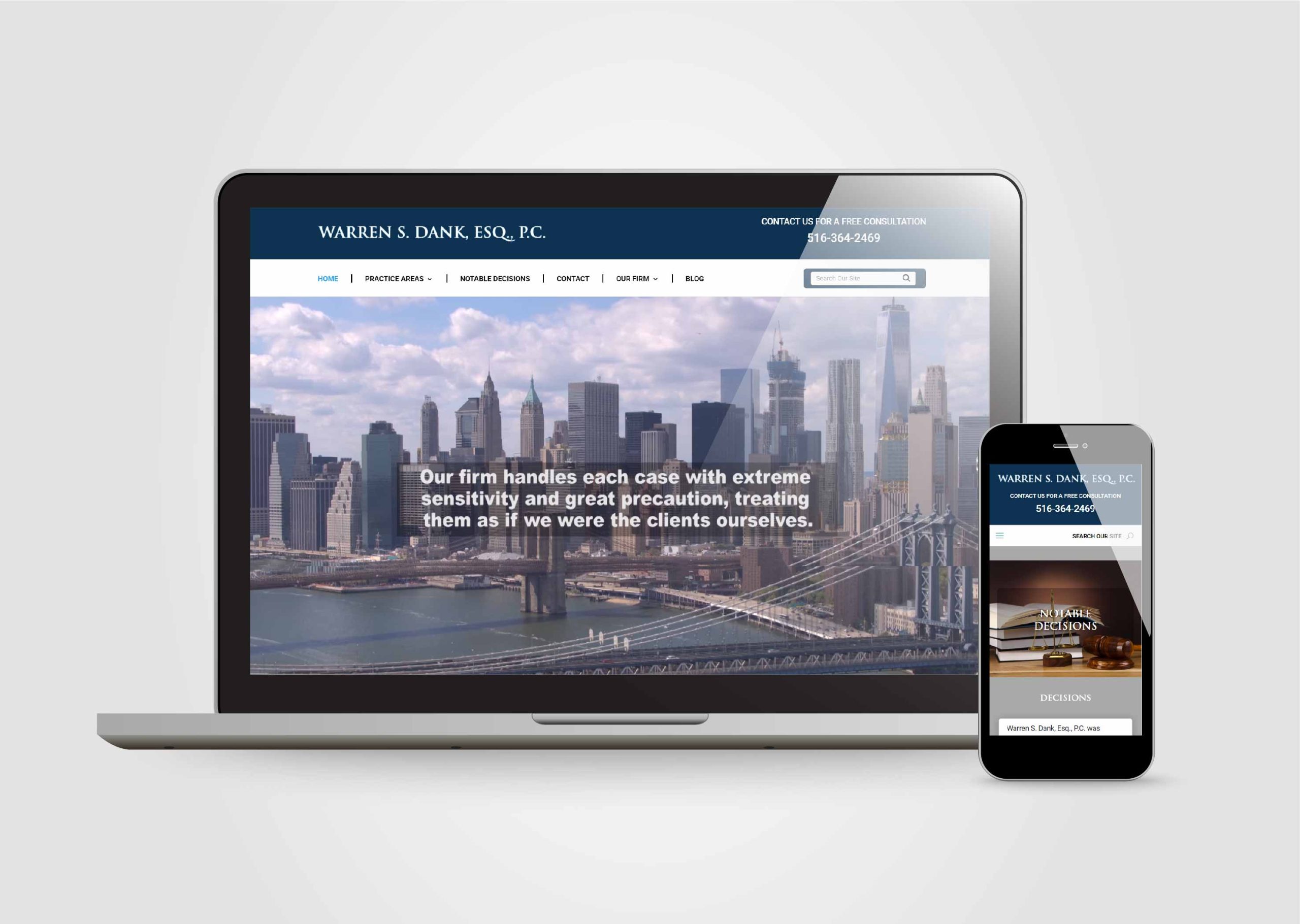This image showcases a silver-bodied laptop with a black-bezel screen, alongside an upright smartphone, both displaying the same website. On the laptop screen, the website header reads "Warren & Dank, ESO and PC" in the top left corner, with a navigation bar below featuring tabs labeled "Practice," "Media," "Contact," and "Blog." Dominating the center of the screen is a cityscape background with an overlay text that states: "Our firm handles each case with extreme sensitivity and great precaution, treating them as if we were the clients ourselves." To the right, the smartphone mirrors the same website, albeit with part of the display obscured, showing the phrase "decision" among some partially visible text.